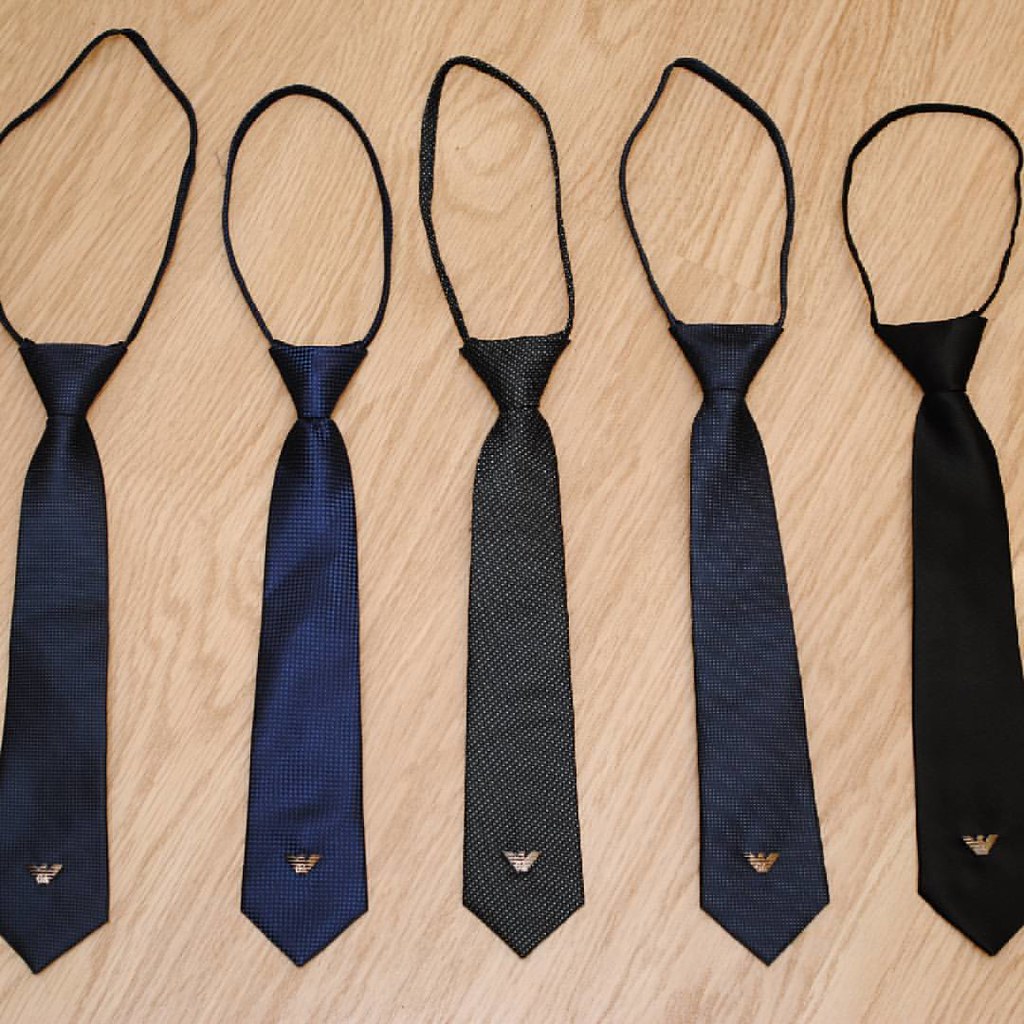A color photograph depicts five pre-tied neckties neatly arranged on a diagonally grained, maple-colored board, which might be a laminate wood floor. The ties appear to be various shades of blue and black, ranging from deep, almost black blue to different hues of navy and royal blue. Each tie is equipped with an elastic band that allows for easy wearing without the need to retie them, ideal for young boys, possibly for a formal occasion like attending a boarding school.

At the top of each tie is a neatly formed knot, ready to be slipped over the head and adjusted by sliding the elastic band, functioning much like a lasso. The bottom half of each tie bears a distinctive gold emblem or logo resembling a bird in flight, adding a touch of elegance. The ties exhibit a similarly textured finish, with some featuring subtle patterns such as diagonal stripes or small white dots, enhancing their refined appearance.